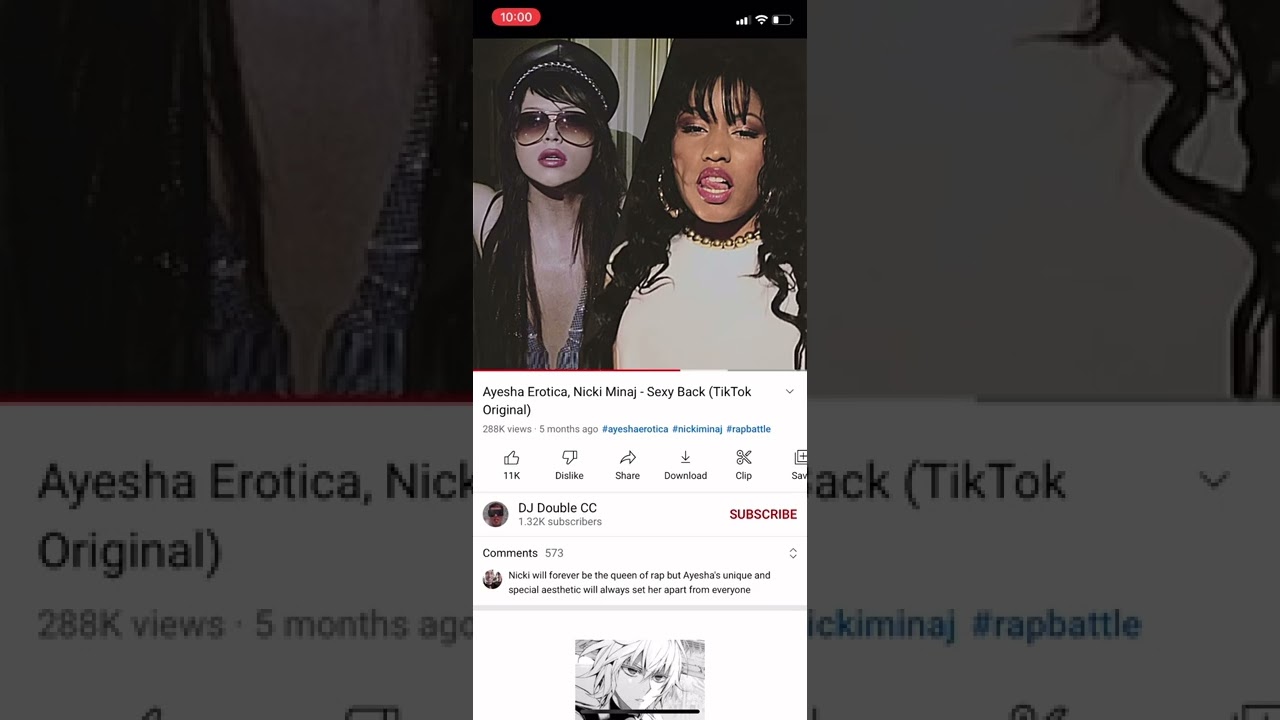Here is a descriptive caption:

"A YouTube screenshot titled 'Aisha Erotic - TikTok Original' is displayed. In the background, a larger YouTube channel interface is visible, suggesting a significant viewership or subscriber base. The screenshot features a woman wearing glasses, who appears to be singing a song related to Nicki Minaj. The standard YouTube mobile interface is apparent, complete with share buttons and other typical navigation elements. The image captures the essence of a vibrant and engaging content piece shared on the platform."